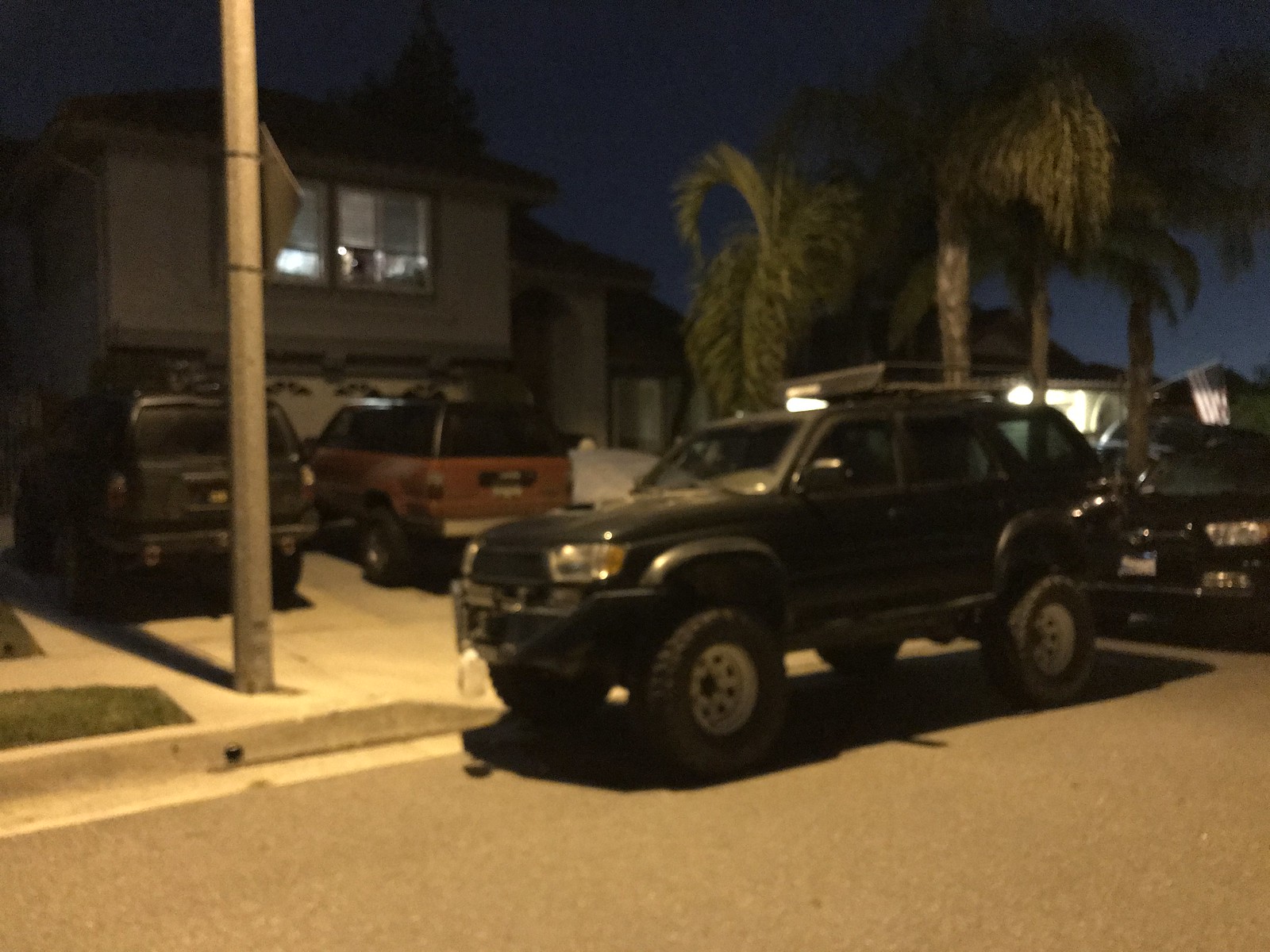The image depicts a nighttime scene outside a two-story house, likely located in a neighborhood with a warm climate such as California or Florida, evidenced by the presence of short, yet wide, palm trees in the front yard. The house has a light gray exterior with decorative brickwork around the garage, which has its door closed. The scene is predominantly illuminated by a yellow-tinged streetlight casting its glow over the area, giving the photo its distinct color tone.

Several vehicles crowd the driveway and street. In the driveway, there is a black car and a red car with a black top, while a vehicle draped in a cloth cover is also present. Blocking these cars from exiting the driveway is another vehicle parked across it, accompanied by additional vehicles including a black Jeep and another black car parked along the street. Notably, the neighborhood features well-maintained lawns, with the grass neatly cut.

Visible through the windows above the garage, lights are on in what might be two bedrooms, with shades partially drawn, possibly indicating occupants inside. The neighboring house, which is also visible, bears an American flag and has lights on the patio, further contributing to the nighttime atmosphere. A telephone pole with a sign adds to the suburban street's details, framing the scene captured from an angle across the street.